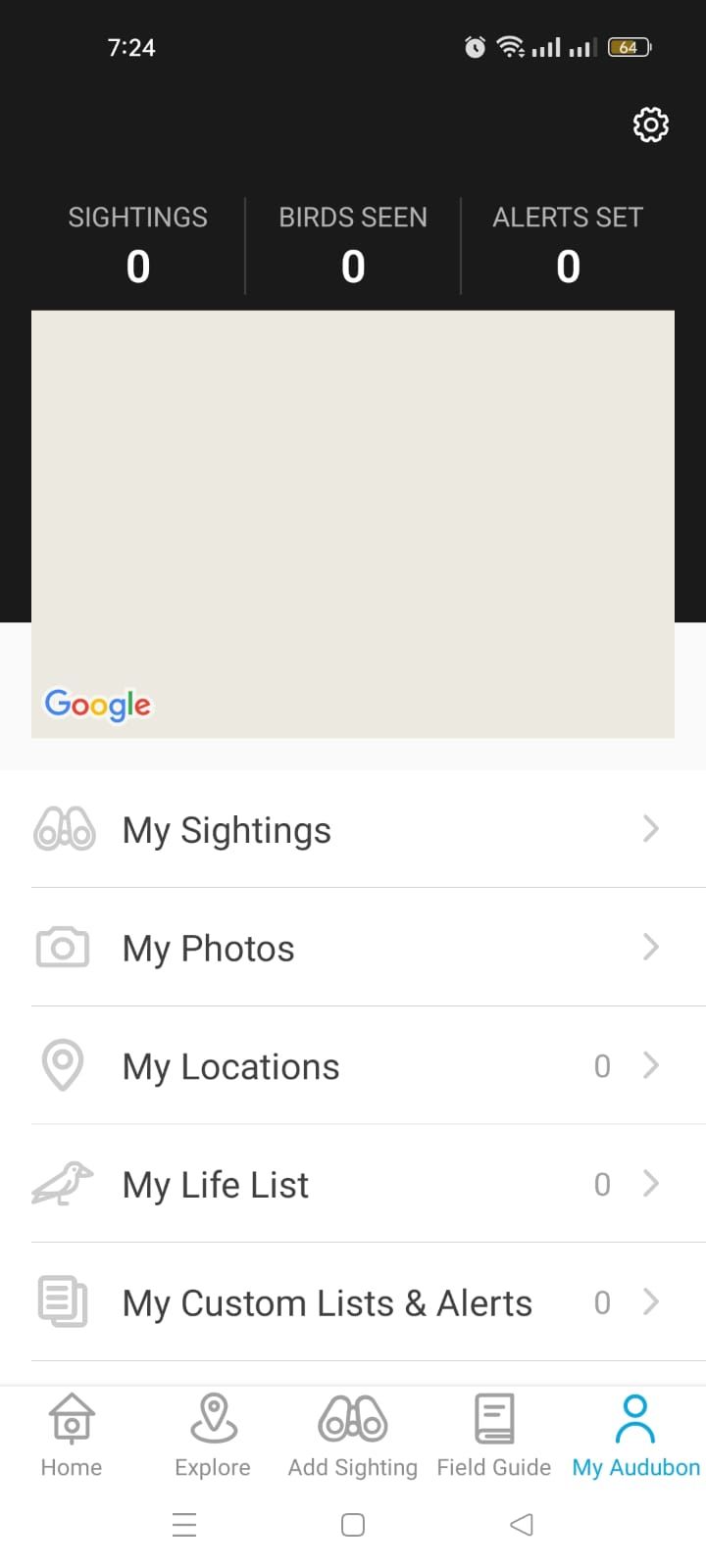A detailed screenshot of a birdwatching mobile app interface taken at 7:24 AM. At the top of the screen, typical status icons are visible on the right: an alarm clock, Wi-Fi signal strength, mobile network signal strength, an unidentified icon, and battery level at 64%. The app's interface includes a settings button (gear icon) located at the top right corner, which is part of the app’s design. 

The main section of the screen shows various statistics: "Sighting: 0," "Birds seen: 0," and "Alert set: 0." Below these, a Google Map area appears, although currently blank. 

Underneath the map, there are several clickable options: "My Sightings," "My Photos," "My Locations: 0," "My Life Lists: 0," "My Custom Lists and Alerts: 0." 

At the bottom of the screen, there is a navigation menu with five tabs: "Home," "Explorer," "Add Sighting," "Field Guide," and "My Audubon," with the "My Audubon" tab currently selected.